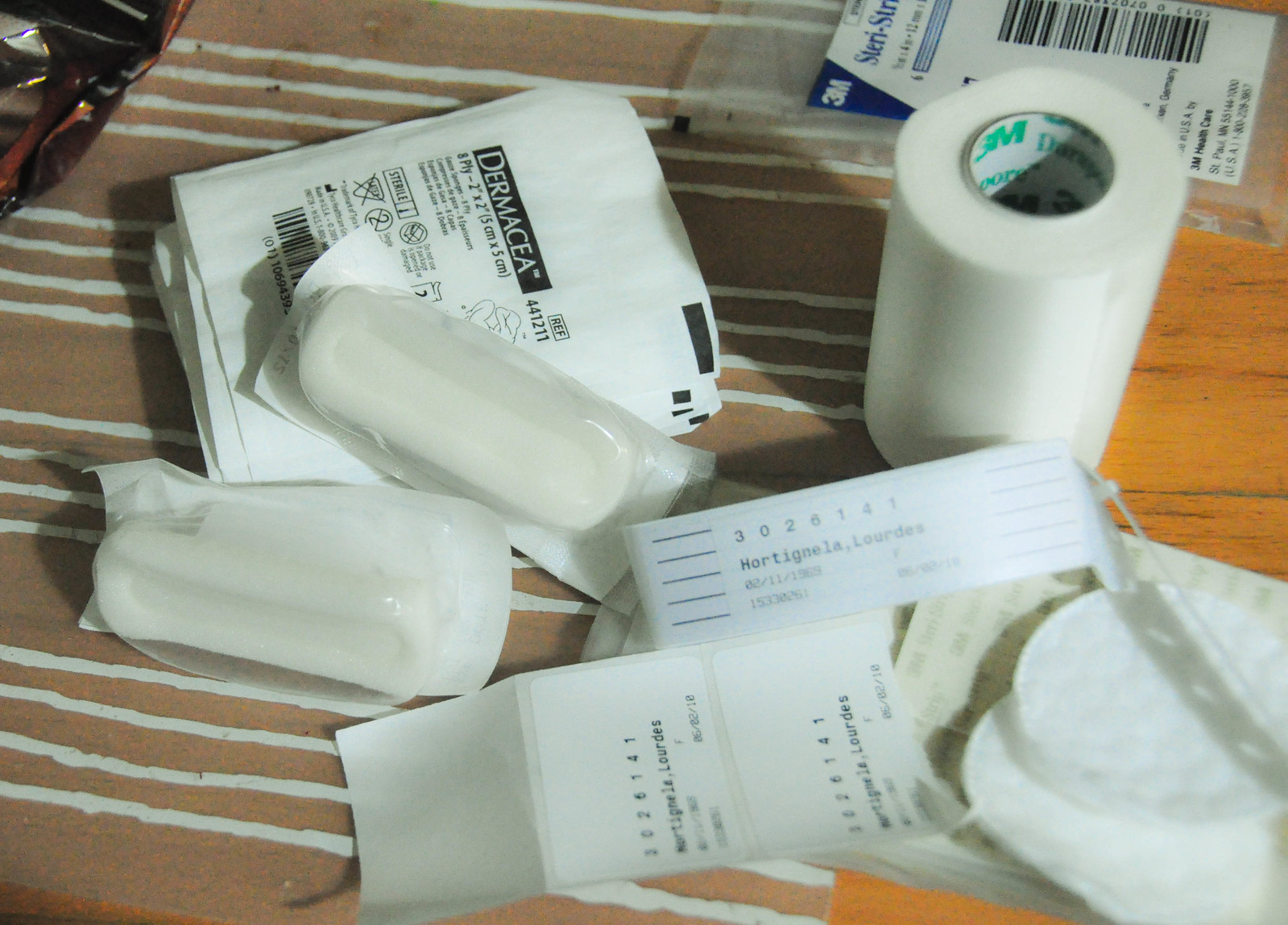This is a detailed, color photograph of a collection of medical supplies arranged on a wooden table. The majority of the items are placed on a brown placemat with horizontal white stripes. Among the visible supplies is a roll of white medical tape, identifiable by the core that reads "3M." Nearby, there's an empty clear package labeled "3M Steristrips" partially visible at the top right corner. A hospital ID bracelet is prominently featured near the middle, with the text "HORTIGNELA Nella Lourdes, 02-11-1969, F-1533-0261, 3026141" clearly printed on it. Underneath the bracelet, two stickers display the same identifying information. To the bottom right, there's a small stack of round cotton pads. Two unclear, wrapped medical items are positioned near the left of the center, adjacent to a partially visible package labeled "DERMACEA." The overall scene suggests a focus on wound care materials spread out in a somewhat organized manner.